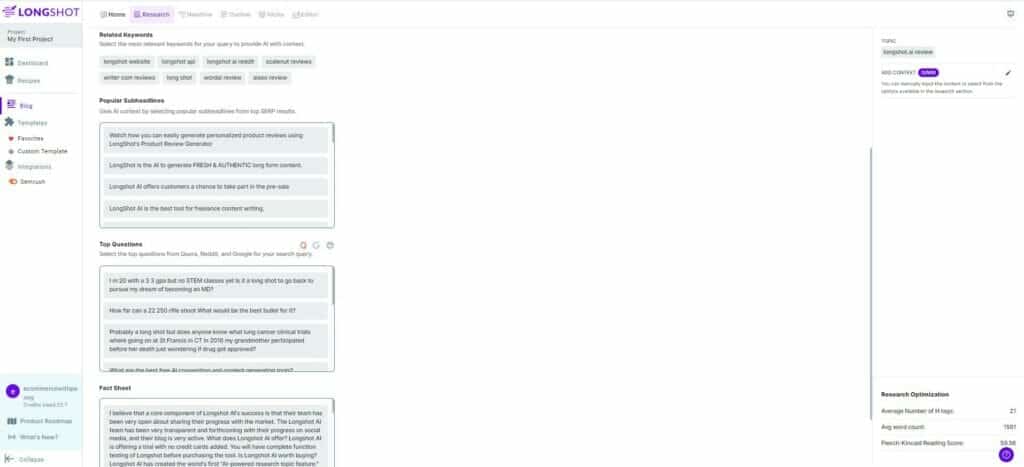The image depicts a user interface page, likely from an educational or documentation website designed to assist in writing scientific papers by consolidating various resources. The left side of the screen shows a laptop, perhaps displaying a final project. The page itself features an "Experiment Abstract."

At the top, there are tabs labeled "Related Keywords," and "Popular," along with a section titled "Top Questions." The right side of the interface shows a scroll bar leading to a chatbox module, which includes highlighted topics and an edit bar with an edit icon on the right. Additionally, there is a purple notification next to this functionality.

At the bottom of the screen, the interface lists "Recent Organizations" and possibly some averages or statistical numbers, likely reflecting data or stats relevant to the scientific paper or channel.